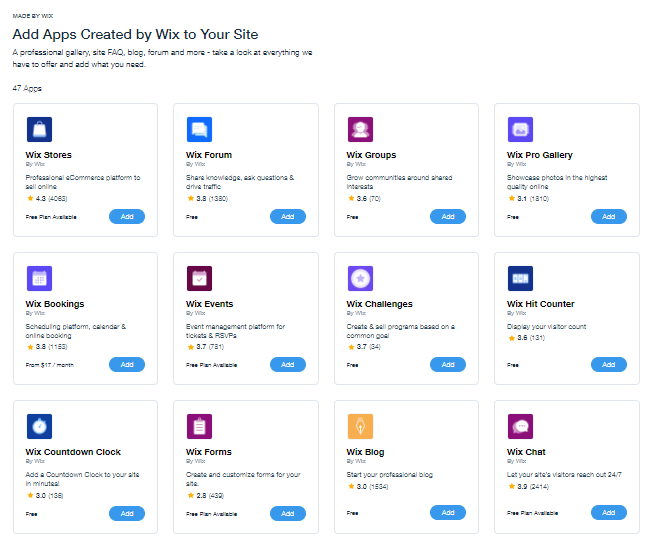The image is a landscape-oriented rectangle with a predominantly white background. In the upper left-hand corner, the phrase "made by WX" is written in black. Just below, in a larger font, it reads, "Add apps created by WIX to your site." Returning to a smaller font size, the text continues, "A professional gallery, site FAQ, blog, forum, and more. Take a look at everything we have to offer and add what you want."

As you move further down the image, there is mention of "47 apps," followed by a structured matrix of squares bordered by thin gray lines. Each square contains different widgets or apps available for integration. For instance, the first square showcases a white shopping bag icon within a blue square, labeled "WIX Stores," accompanied by the description, "Professional e-commerce platform to sell online." Below this description is a review rating of "4.3 out of 5 stars," and a blue oblong button that says "Add." Each app in the matrix features similar details including icons, descriptions, ratings, and "Add" buttons.